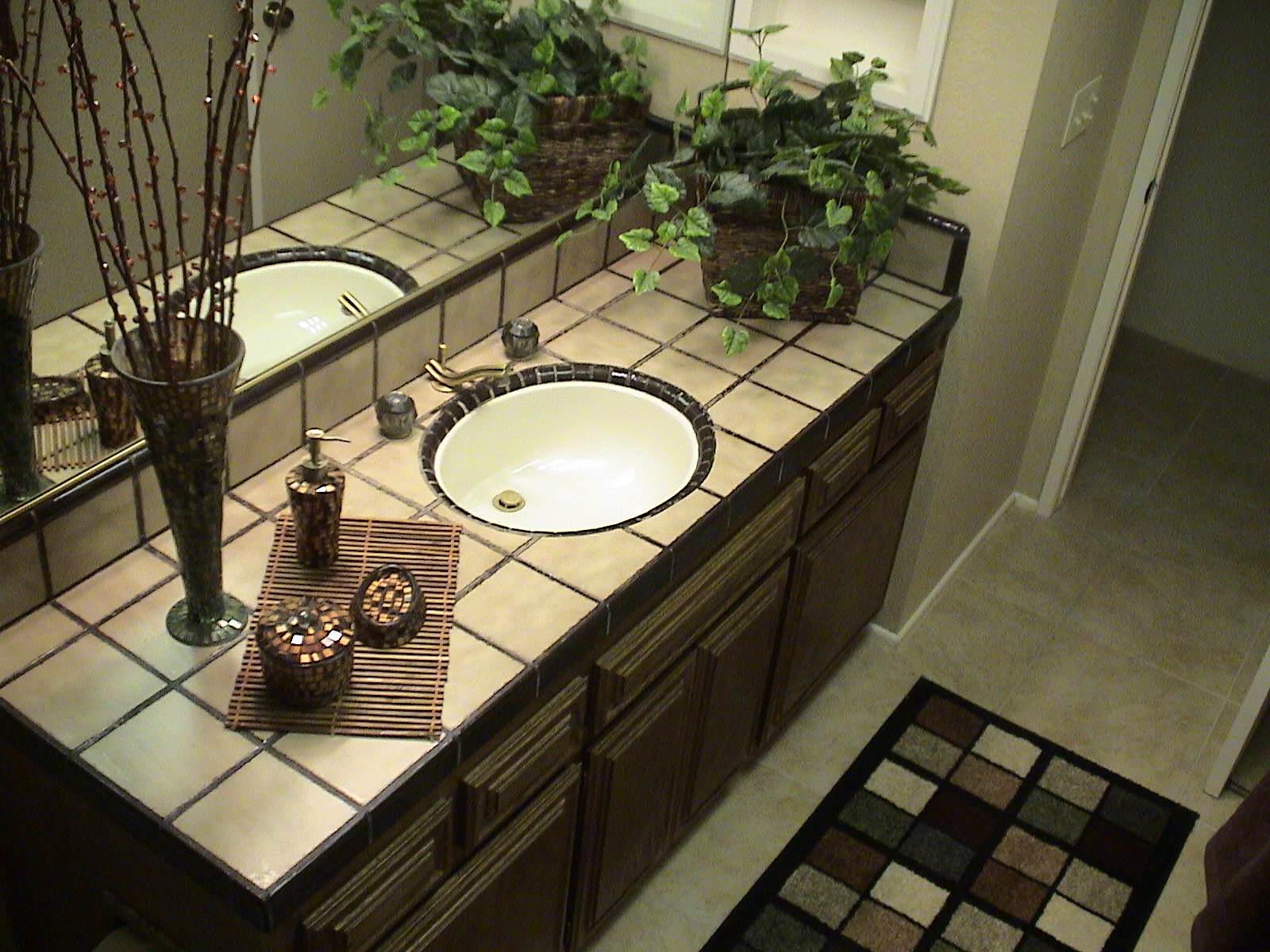This indoor color photograph captures a detailed overhead view of a bathroom countertop and sink area. The countertop is composed of square tan tiles with brown grout lines, and prominently features an underhung white porcelain sink. Centrally positioned above the sink is a golden faucet flanked by matching knobs on either side. 

To the right of the sink, at the far end of the countertop, sits a basket filled with artificial green foliage. In the foreground on the left side, a tall vase adorned with thin vertical sticks decorated with sparkling jewels adds an elegant touch. In front of the vase rests a wooden mat, which holds a few items: a powder dish, a soap dish, and a soap dispenser.

The bathroom mirror is aligned with the backsplash, capturing and reflecting the various objects on the countertop. On the lower right corner of the image, the white tile floor is partially visible, along with a multicolored area rug situated directly in front of the sink. This rug features a symmetrical pattern composed of red, white, light tan, and black rectangles.

Beneath the sink, there are wooden raised panel cabinets without visible door pulls or knobs. In the background on the right, part of a door leading to a hallway is noticeable. The photograph is devoid of any text or captions, allowing the visual elements to speak for themselves.